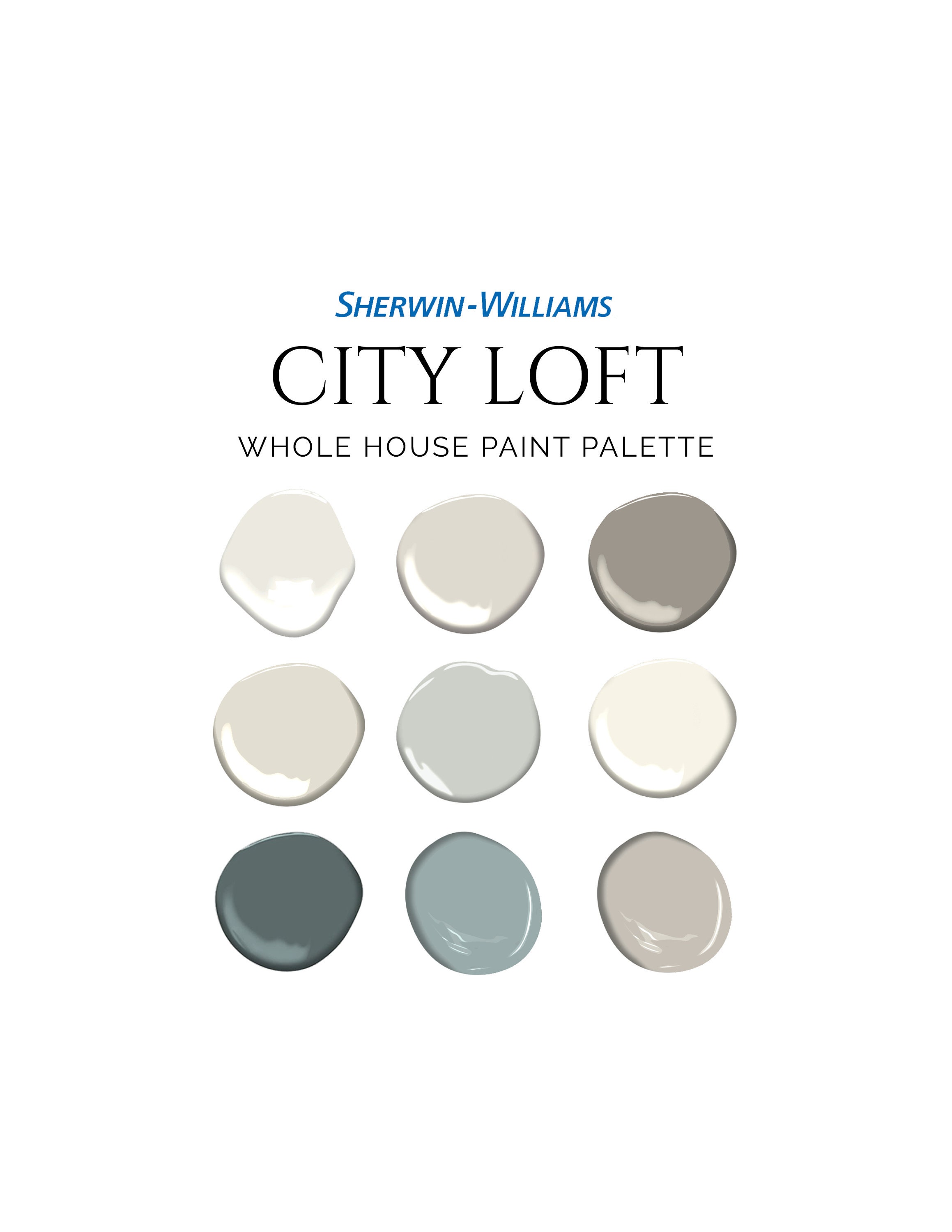The image depicts an advertisement for the Sherwin-Williams "City Loft" Whole House Paint Palette. At the top, the recognizable Sherwin-Williams logo is prominently displayed. Below the logo, the text reads "CITY LOFT" in large black capital letters, followed by "WHOLE HOUSE PAINT PALETTE" in slightly smaller black capital letters. The focal point of the image is a grid of nine circular matte paint samples, arranged in a 3x3 pattern. These samples showcase a gradient of colors, starting from various shades of off-white through gray to darker hues. 

In the top left corner, the first sample is a light off-white, bordering on ivory. Adjacent to it is a taupe shade, followed by a grayish-brown hue on the top right. The middle row starts with a light cream color to the left, transitions to a medium taupe, and ends with a distinct cream color on the right. The bottom row presents a dark steel gray on the left, a medium to dark gray in the center, and a subdued, rosy color on the right. Each sample exhibits a nuanced variation in tone, collectively forming an elegant and cohesive palette suitable for whole-house applications.